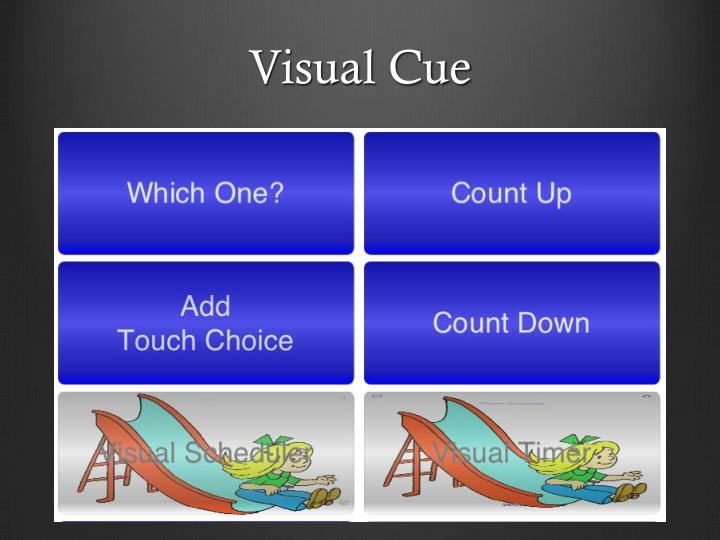The image appears to depict a graphic, potentially from a PowerPoint presentation or an interactive educational game, set against a gray background. Dominating the top of the image in thin white font is the title "visual cue." Directly below this, there is a neatly divided white box featuring six sections separated by white lines. The top four sections have blue backgrounds. The top left section reads "which one?" and the one below it states "add touch choice." The top right section says "count up," while the one below it says "count down."

At the bottom of the image, on either side, are two illustrated buttons depicting a little blonde girl with a green bow in her hair, sliding down a red slide with a blue metal surface. She is donned in a green shirt, blue jeans, and brown shoes, and is captured in a sitting position with arms beside her, smiling and looking slightly to the left. Between these illustrations, in thin gray font, are the labels "visual scheduler" on the left and "visual timer" on the right. The color scheme includes shades of gray, blue, white, orange, red, green, yellow, and light blue, suggesting an interactive, playful, and educational design.